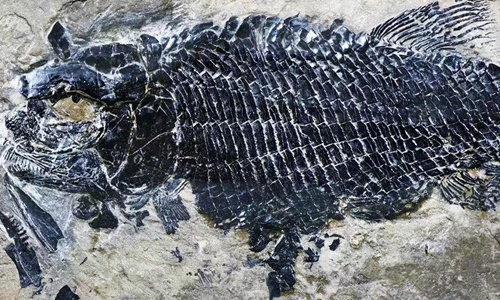The image appears to be a highly detailed drawing or painting of a fossil-like creature, resembling a prehistoric fish with some unusual features. The creature occupies approximately 80% of the picture, with what looks like a rock texture in the background, enhancing the fossil impression. Its body is elongated and covered in scales similar to those of a crocodile or an alligator. On the top right, a dorsal fin is visible, and towards the lower part of the body, there is a fin indicative of its aquatic nature.

The head, positioned to the left side of the image, has distinct features that set it apart. It has an unusually large, wide eye with a small black pupil, which might suggest a mix between fish and other animal characteristics, somewhat reminiscent of a cat. This eye is strikingly yellow with the black pupil. Additionally, the head includes two very small ears, further adding to its peculiar appearance. The absence of text and the overall decrepit, old-looking condition of the illustration contribute to the impression that this could either be a depiction of an ancient fossil or a crafted artistic representation intended to emulate the discovery of such an artifact.